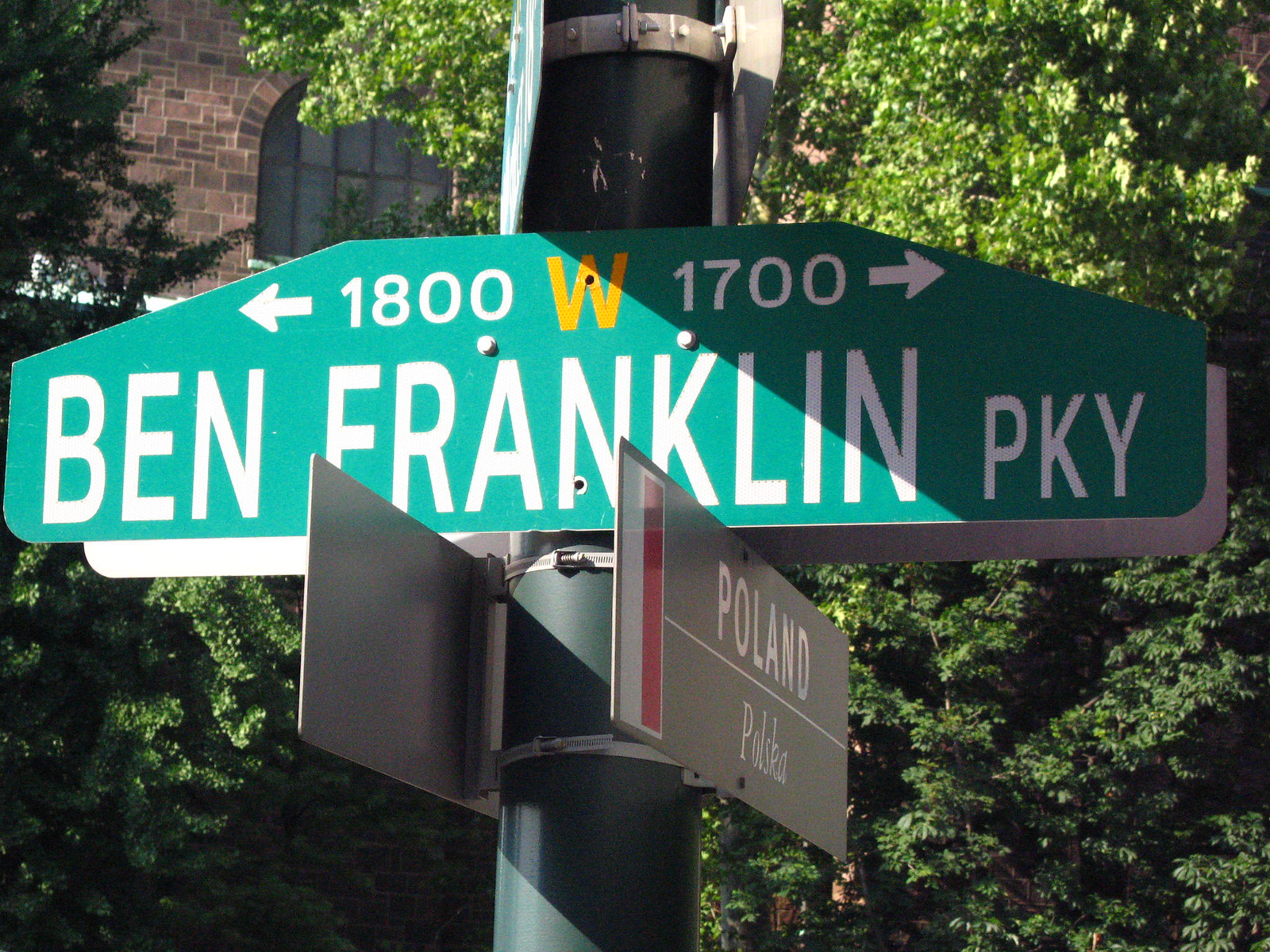A close-up photograph captures a street sign on a sunny day. On the right side, the top corner of the image is adorned with the sunlit leaves of a green deciduous tree, giving them a lighter green hue. To the left, a stone building made of pinkish-gray stone features a charming arched window. The street sign, positioned prominently, stands out as the focal point against the greenish backdrop. 

The sign is rectangular with slight upward extensions on each side, becoming narrower at the top. The top line of the sign features a left-pointing arrow followed by the number "1800" and a gold "W". An arrow pointing to the right displays the number "1700" in white lettering. Below, in capital letters, the sign reads "BEN FRANKLIN PKY." 

Partially obscured behind this prominent sign is another street sign, visible only by its gray pole, but its text is indiscernible. Beneath the main sign, oriented in an opposite direction, is a gray sign with white letters reading "POLAND" and an inscription in another language below it.